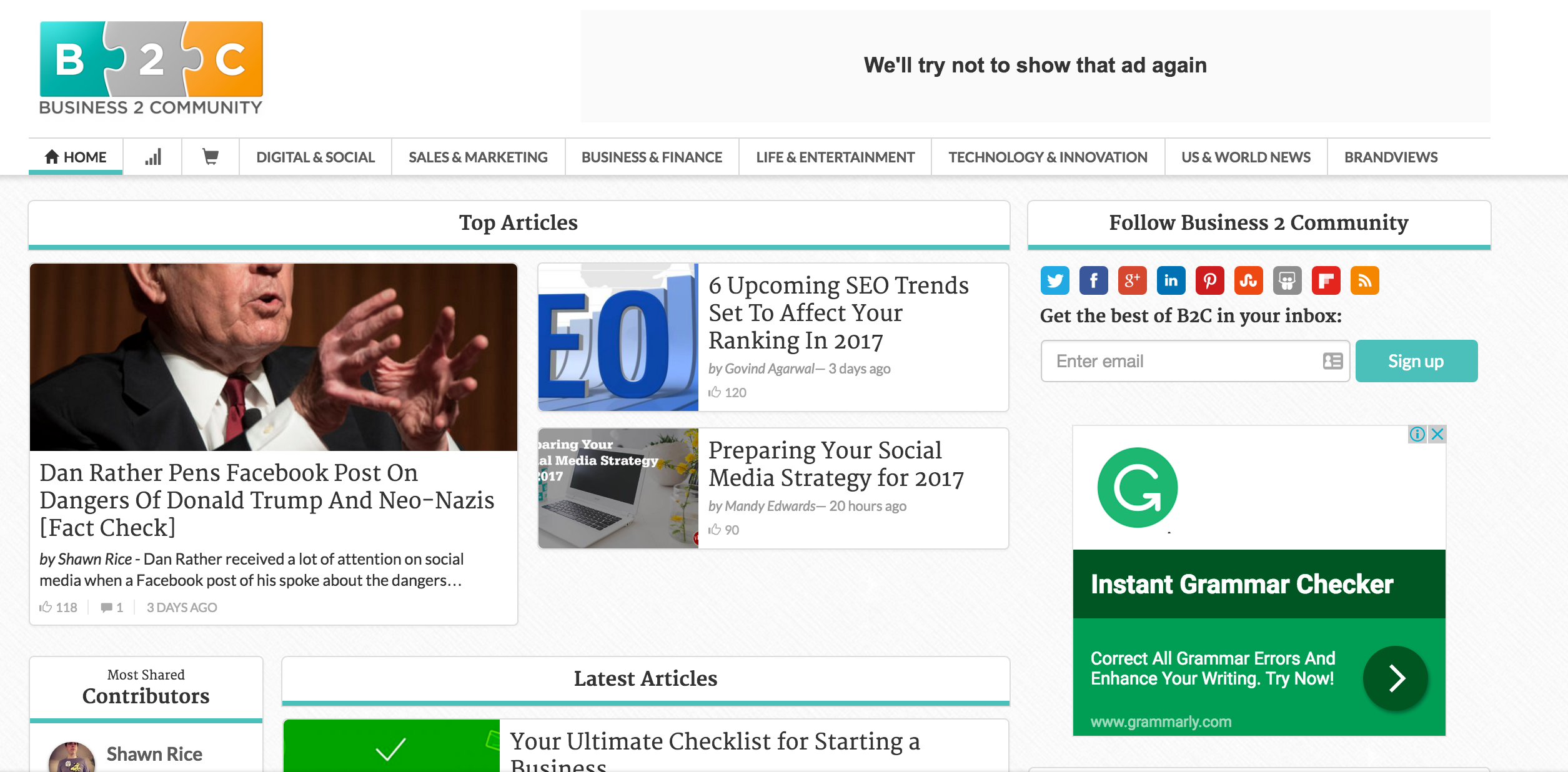This detailed image portrays a website interface for "Business to Community" with a prominent header featuring three interlocking puzzle pieces. The first puzzle piece is turquoise blue with a white, capitalized letter "B" inside. The second piece is gray with a white number "2", and the third piece is light orange containing a white, capitalized letter "C". 

The phrase "Business to Community" is displayed prominently on a white background underneath these puzzle pieces. The central section of the page features a light gray background with a notification reading, "We'll try not to show the ad again".

Beneath this, on a white background, there is a navigation bar with various options spanning from left to right. These options include: "Home" (highlighted with a turquoise blue underline), an icon indicating Wi-Fi or cell signal strength, and a shopping cart icon. The navigation menu extends to include categories such as "Digital and Social", "Sales and Marketing", "Business and Finance", "Life and Entertainment", "Technology and Innovation", "U.S. and World News", and "Brand Views".

Further down, in black print, it says "Top Articles". Adjacent to this is a call-to-action to follow "Business to Community" on various social media platforms. Below it reads "Get the Best of B2C in Your Inbox" with a field to input your email and a teal-colored "Sign Up" button.

The left-hand section lists top articles, including titles such as "Dan Rather Penn's Facebook Post on Dangers of Donald Trump and Neo-Nazis," "Fact Check: Six Upcoming SEO Trends Set to Affect Your Ranking in 2017," and "Preparing Your Social Media Strategy for 2017."